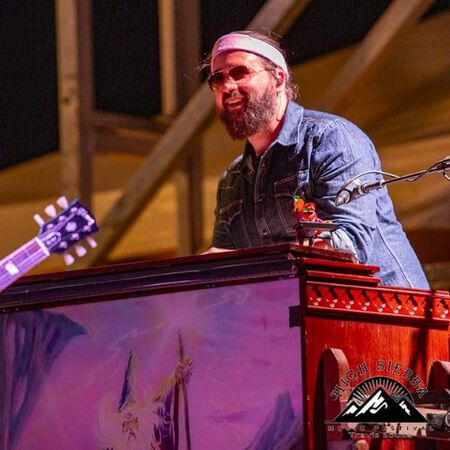This detailed photograph captures a man with a full beard and mustache, standing confidently on a stage behind an ornate podium. He is dressed in a blue jean jacket and has a cloth headband tied around his brown hair. His eyes are shielded by small, wire-rimmed, dark sunglasses. Resting beside him is a microphone angled toward his direction, suggesting he is about to speak or perform. The podium he stands behind is vividly painted with a wizard and a castle set against a pink background. Additionally, there's a distinctive emblem on the lower right corner of the podium showcasing the Sierra Mountains symbol. To the left of the man, the top of an electric guitar is visible, hinting at a musical performance. Behind him, tall wood timbers reminiscent of a stage setting add a rustic backdrop to the scene.